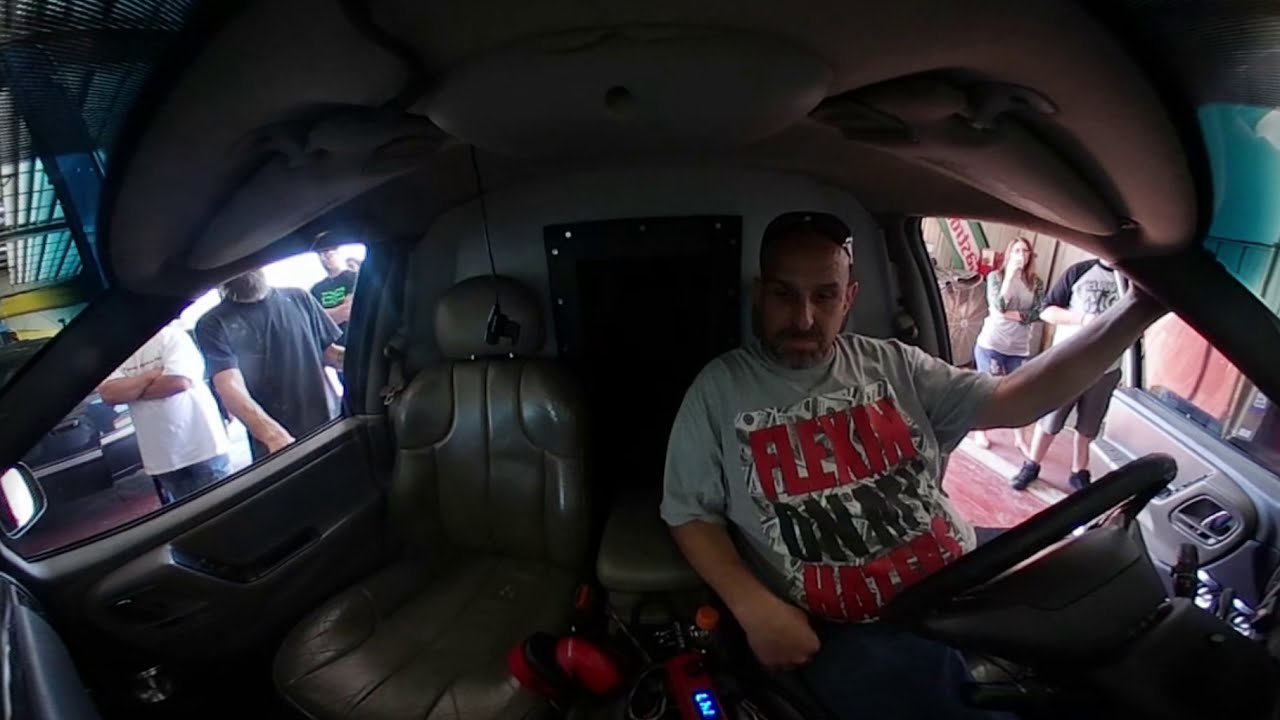This color photograph, taken with a wide-angle lens, captures the detailed interior of a black leather-seated car at a show. The vehicle features sculpted seats with red accents, possibly indicative of a stock car's interior. Central to the image is a man in his 40s, with a brown beard and mustache, wearing a gray t-shirt that reads "Flexin' on My Haters" in red, black, and white letters. He is seated behind the steering wheel, looking towards the center console and facing the camera. Sunglasses rest atop his head. The image, set in a daytime retail area, shows a somewhat dimly lit car interior. Out the driver's side window on the right, two young adults in their 20s, dressed in t-shirts and blue jean shorts, stand on a sidewalk gazing into the vehicle. On the left side, seen through the passenger window, two men—one with crossed arms—also observe the car. The photograph is horizontally oriented, and the man, slightly to the right of the center, anchors the composition, highlighting the dynamic between the vehicle's interior and the curiosity of onlookers outside.